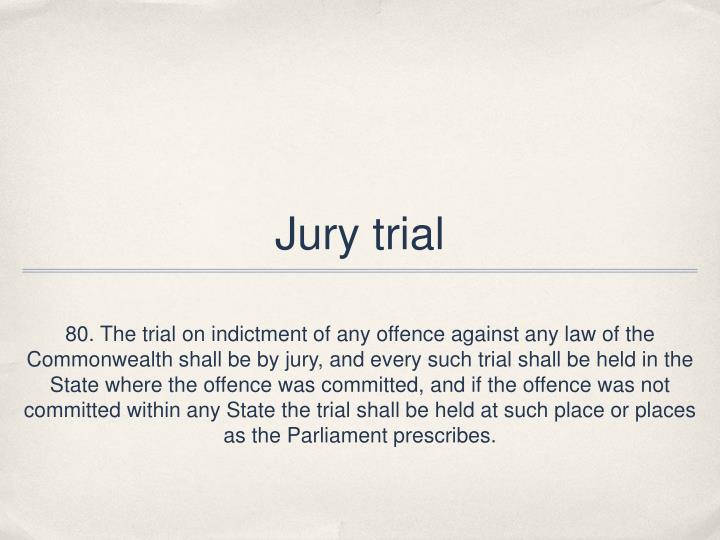The image features a text excerpt on a white background, seemingly from either a PowerPoint presentation or a legal document. The top portion of the page is blank, followed by the bold, navy blue title "Jury Duty". Directly beneath the title, two thin horizontal lines span almost the entire width of the page. Positioned below this, the text begins with "80." in a distinct line, leading into a detailed legal statement: "The trial on indictment of any offense against any law of the Commonwealth shall be by jury, and every such trial shall be held in the state where the offense was committed, and if the offense was not committed within any state, the trial shall be held at such place or places as the Parliament prescribes." This definition pertains to the procedural conduct of jury trials within the Commonwealth, indicating jurisdiction based on the location of the offense. The overall layout suggests it may be a segment from a law book or educational material on legal practices.